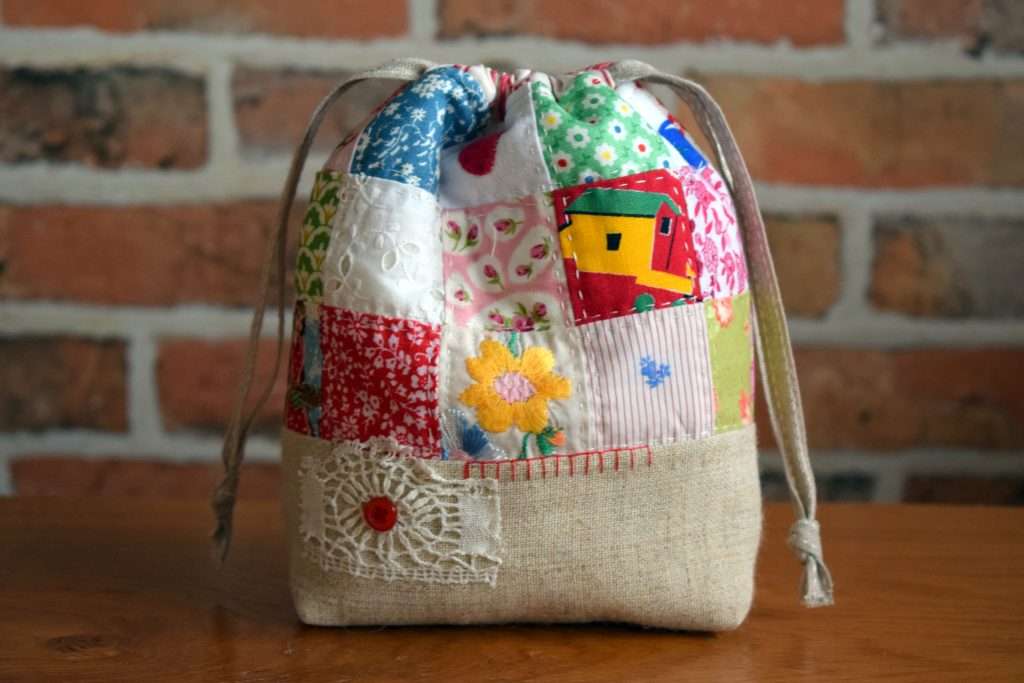In this indoor photographic image, a handmade canvas bag is artistically displayed on a wooden table against a backdrop of thickly mortared orangey brick walls. The bag is skillfully crafted with two fabric handles and distinct patchwork detailing, which makes it a unique piece. The bag features three rows of decorative squares, reminiscent of a quilt. These squares include a combination of embroidery and sewn-in fabric designs. 

The top row features various patterns: blue backgrounds with white flowers, white backgrounds with red blots, an assortment of red, yellow, and green floral designs with white petals on green backgrounds, an image of a schoolhouse or barn in yellow and green on a red background, intricate roses, and embroidered floral shapes. One square has a mini print of white flowers on a red background, alongside an embroidered daisy or sunflower and a striped background with blue plants.

The bottom of the bag showcases an embroidered spider's web with a red center, adding a striking focal point to the piece. Tanned laces accentuate the sides, and a lace patch adorns the tan base of the bag, completing its rustic charm. Each fabric patch on the bag is meticulously stitched, either by hand or machine, emphasizing the detailed craftsmanship of this unique accessory.